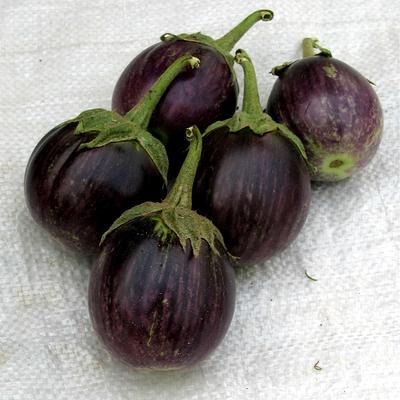The image features five dark lavender, round fruits that resemble smaller, rounded eggplants or large grapes. Each fruit is topped with a bright green stem, resembling a small hat with prongs, and has delicate leaves draping around the stem area. The fruits are arranged closely together on a slightly dingy white paper towel or canvas-like mat. Four of them are grouped on the left side with two in the center, one on top, and one on the bottom, while the fifth fruit is slightly offset to the upper right, touching one from the group on the right. Notably, one of the fruits reveals a tiny dark rim at the bottom, similar to the small indentations found on oranges or apples.